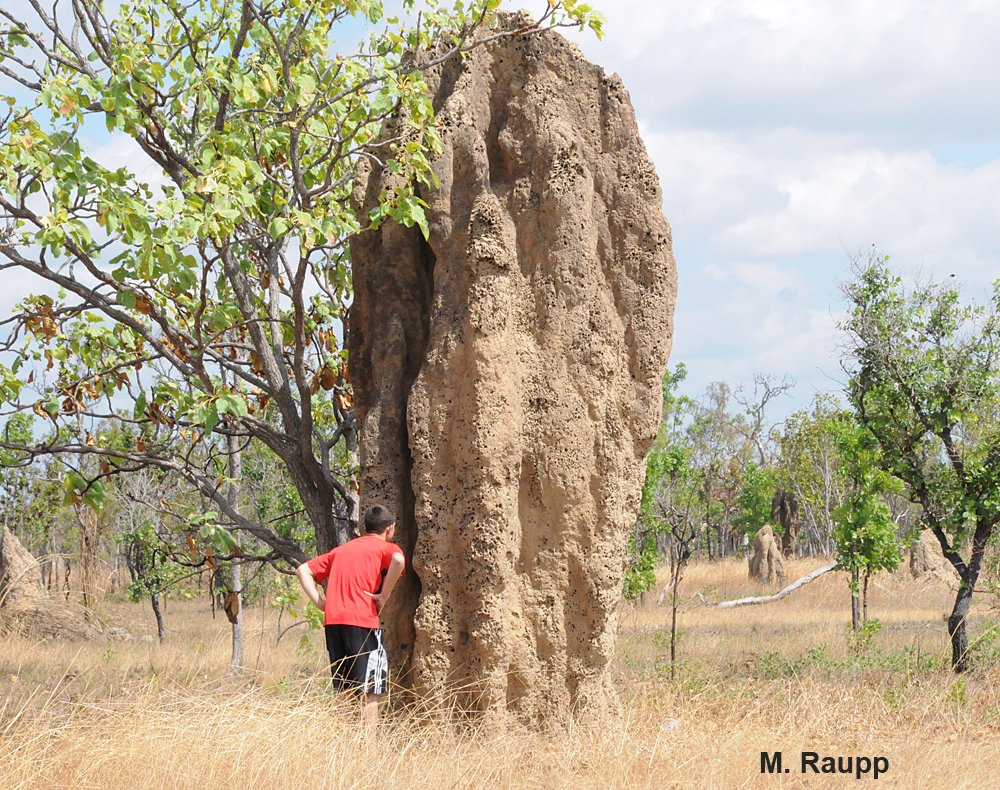In a serene, forest-like area filled with wild, shrubby trees and dry, brownish-yellow grasses, a striking image captures the towering majesty of a unique rock formation. This massive, tan-colored rock juts abruptly from the flat ground, resembling a column with curvy, lumpy sides, and standing nearly as tall as a nearby tree with a small trunk and green leaves. The sky above is a very light blue, dotted with fluffy white clouds.

In front of this geological spectacle, a young boy stands, leaning slightly with his hands on his hips, closely inspecting a crack in the rock. He is dressed in a reddish-orange t-shirt and black shorts with white accents. To the right, another similar rock formation is visible in the distance. This striking photograph is marked with "M. RAUPP" in sans serif black ink at the bottom, suggesting the identity of the photographer.